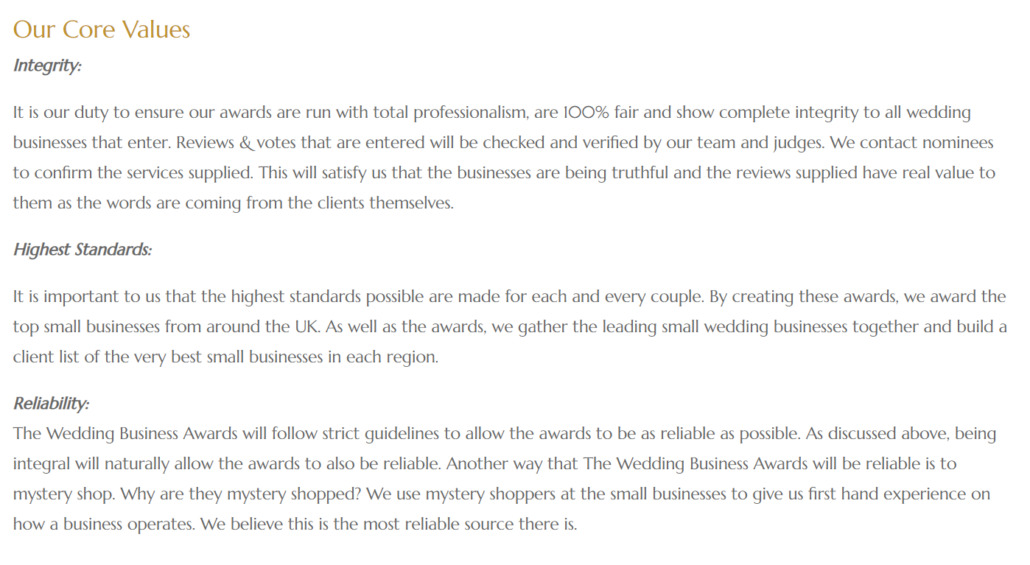In the top left corner of the image, set against a dark yellow background, are the words "Our Core Values." This section is divided into three subcategories: Integrity, Higher Standards, and Reliability.

1. **Integrity:**
   - There are four sentences under this subcategory emphasizing that the awards are conducted with total professionalism, 100% fairness, and complete integrity for all participating wedding businesses. 
   - Reviews and votes submitted are meticulously checked and verified by our team and judges. 
   - We make it a point to contact nominees directly to confirm the services they provided, ensuring the authenticity of the businesses and the real value of the reviews, which come from the clients themselves.

2. **Higher Standards:**
   - This subcategory highlights the importance of maintaining the highest possible standards for every couple.
   - Through these awards, we aim to recognize and celebrate the top small businesses across the UK.
   - By hosting these awards, we bring together leading small wedding businesses, creating a curated client list of the very best in each region.

3. **Reliability:**
   - The final subcategory, Reliability, underscores the strict guidelines that the wedding business awards adhere to, ensuring the awards are as reliable as possible.
   - We believe these guidelines make our awards the most reliable source available.